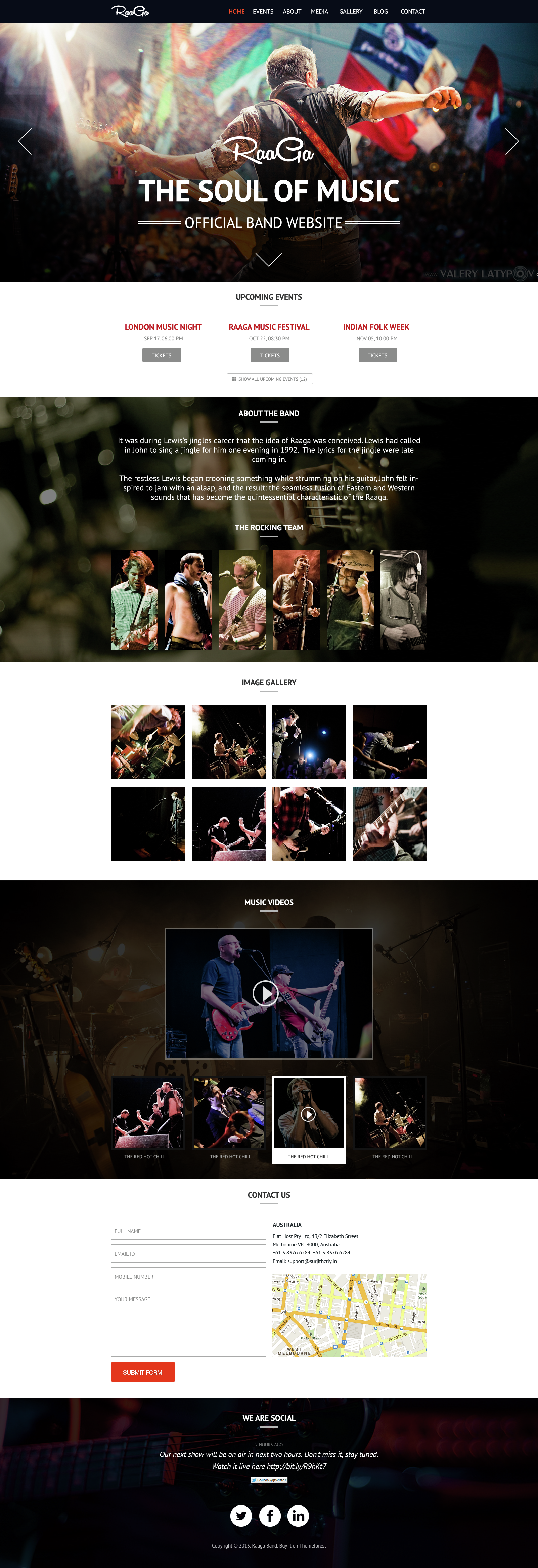The image is a vertically-cropped screenshot, seemingly taken from a phone. At the top, there's a black banner with white text spanning from left to right. Directly below, a photograph captures the back of an individual standing amidst a crowd, with various flags in the background. Prominently displayed is the text "RIAGA, the Soul of Music official band website." 

Beneath this, there are three gray buttons aligned horizontally, each with red text above them—three words in total. The background here is white. Below this section, an area with a blurred image, possibly of someone strumming a guitar, displays white text overlaying it. Following this, there are six photographs arranged showcasing different musicians playing their instruments.

The next section features a white background with eight square photographs, each depicting different band members performing on stage. Moving further down, another section has a background image of someone playing drums and contains an embedded video, likely from YouTube, of two people playing guitars on stage. This video has a play button in its center. Accompanying it are four additional saved videos visible beneath this video.

Further down, the next section has a white background displaying a map with overlaid black text and a form section on the left side featuring a red button with white text. The final segment includes a blurry background that seems to be a close-up of a guitar, white text, and logos for social media platforms Twitter, Facebook, and Indeed. These logos are depicted in white circles with black icons.